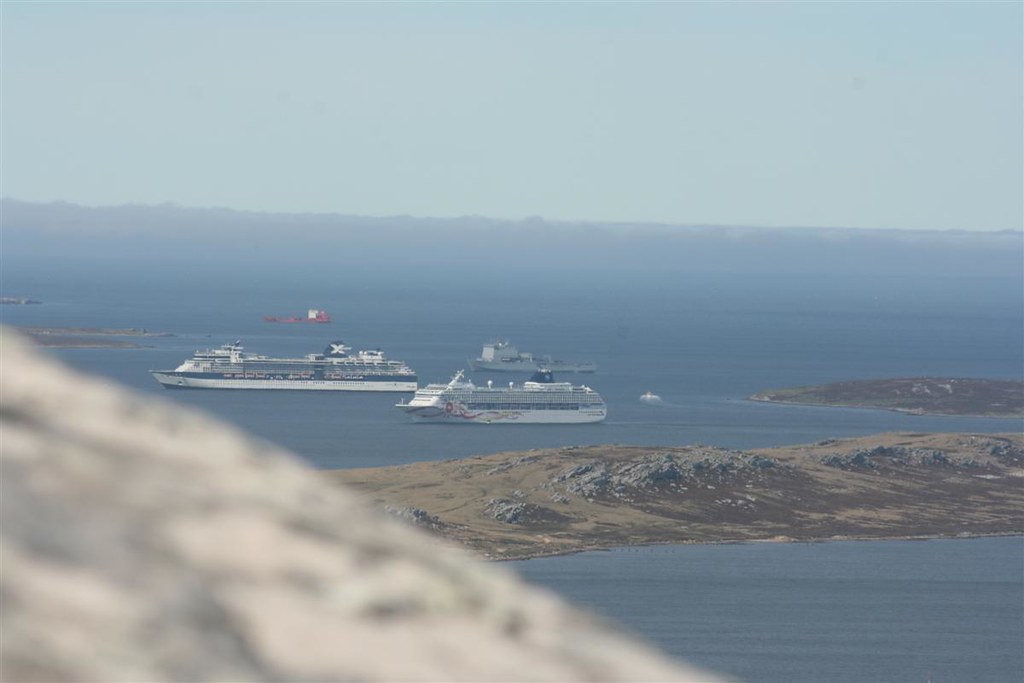This is a color photograph taken from an elevated viewpoint on a hazy day, capturing a wide expanse of the sea that recedes into a clouded horizon. The overall effect of the image is misty and subdued. At the top portion of the photograph, occupying about 20% of the frame, is a light blue sky tinged with smog and clouds. Below the sky, the vast ocean stretches out, appearing still and flat, with a light blue hue that mirrors the sky.

In the distant ocean, there are three large cruise ships or similar vessels. These ships are predominantly white, with distinct designs. One ship features a large horizontal blue line, another displays a red wavy line at the front, and there is a mention of a ship with a tail fin marked by a blue and white X. These ships are situated towards the middle to distant parts of the water.

The lower portion of the image showcases various land masses and rocks. To the bottom left of the image, there is a significant blur, possibly caused by an object partially covering the camera lens. This area includes a close-up of a large, grayish-white rock. Moving towards the bottom right, there are small island-like landforms with rocky outcroppings and multiple hills, colored in a combination of light brown, tan, and mossy green.

Overall, the photograph vividly captures a serene seascape dotted with ships amidst a backdrop of rocky formations and a smoggy sky, blending natural and man-made elements in a misty tableau.